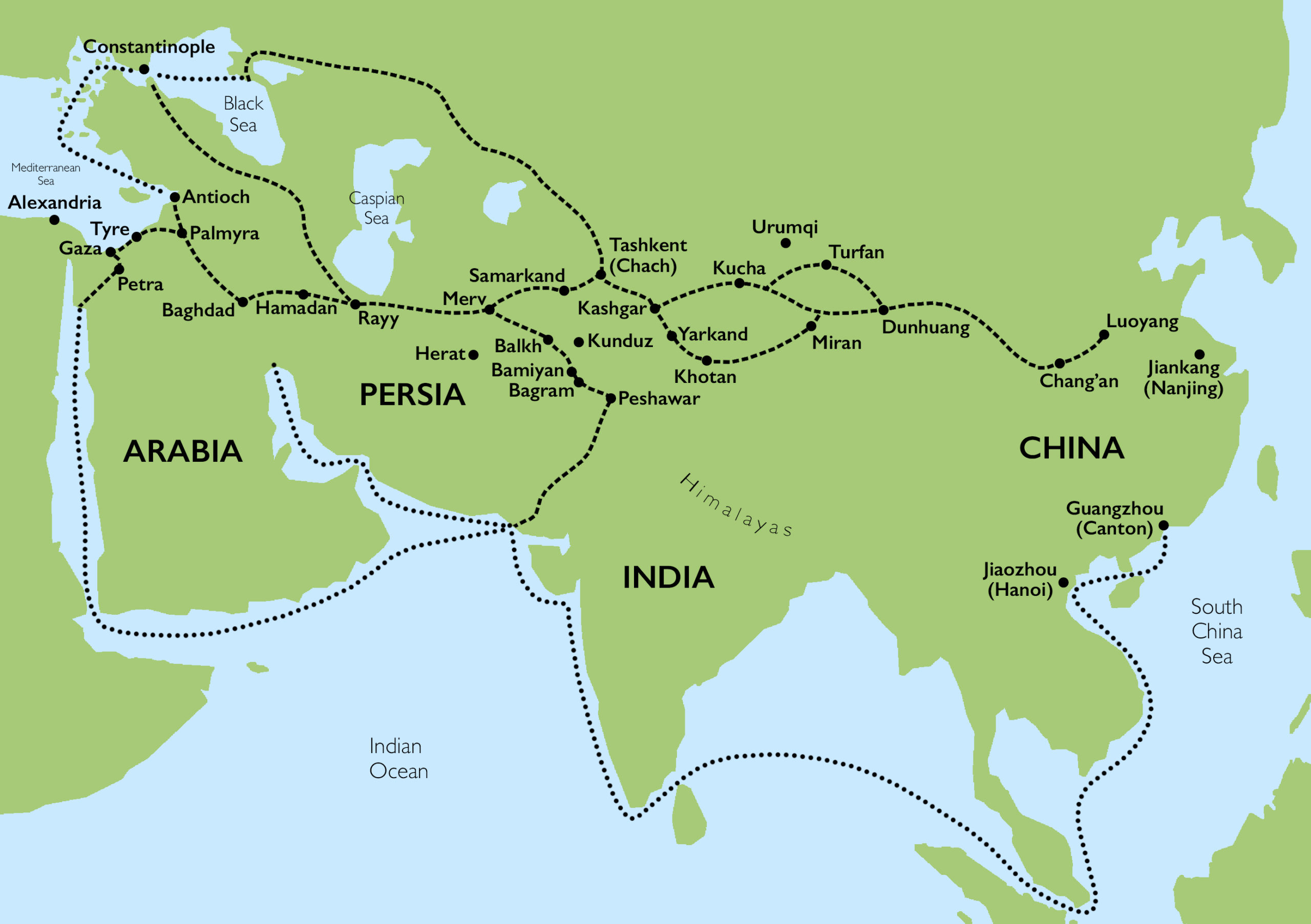This detailed map illustrates the Old World, spanning from China, India, Persia, Arabia, to Constantinople. The map is dominated by flat green landmasses, each labeled with country names and specific cities. Prominent countries include China, located in the top middle-right; India, positioned in the bottom middle; Persia, situated in the middle-left; and Arabia, found right after Persia. At the top of the map, Constantinople is clearly marked. The territories are encompassed by a dotted line, indicating extensive regions of Asia and the Middle East, including the Caspian Sea, the Black Sea, and the Mediterranean Sea at the northern edge, and the Indian Ocean and South China Sea at the southern edge. 

The cities marked along the map create a historical route, likely representing the ancient spice road during the BC times. Key cities include Constantinople, Alexandria, Tyre, Gaza, Petra, Antioch, Palermo, Baghdad, Hamadan, Riyadh, Merv, and Samarkand in the western and central areas, extending to Longzheng, Junkan, Chaten, Guangzhou, Jiangsu in China. Despite the map's sparse detail, these labels, and the flat green color dominant in the geographic areas, provide a clear yet minimalistic representation of the ancient world.